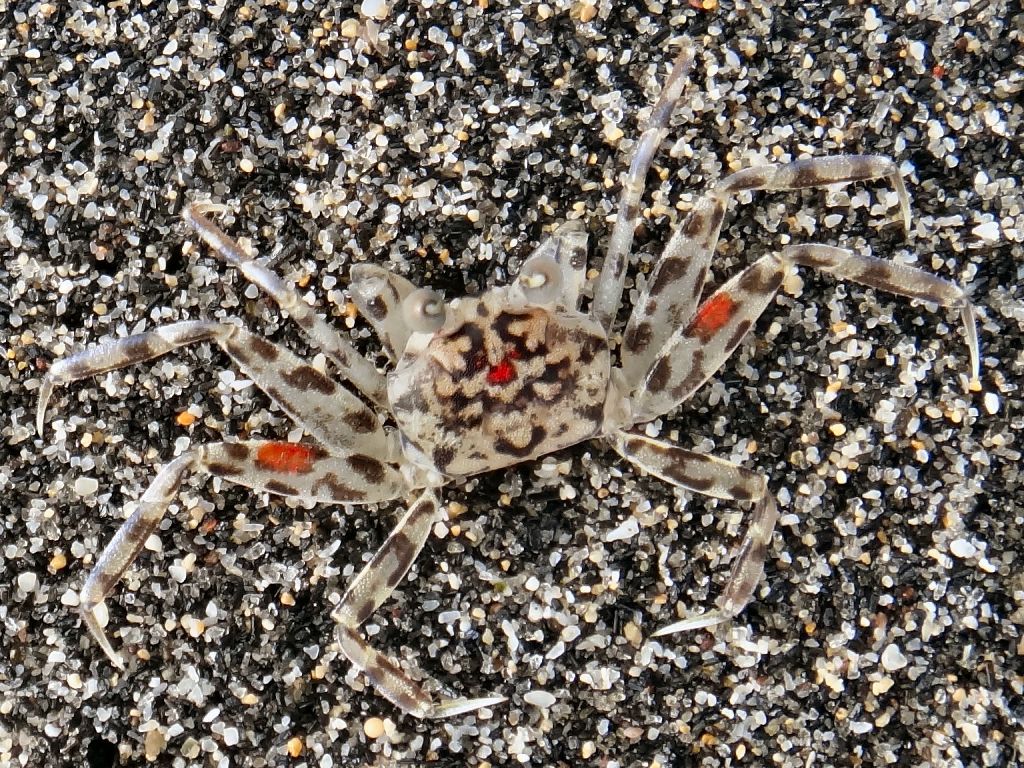This is an overhead photograph of an exotic-looking crab set against a backdrop of small pebbles that almost appear like fine sand, consisting predominantly of black and grey hues intermixed with white, beige, and shades of brown. The crab’s body is a striking grey-silver color adorned with black markings and hints of red that create an interesting pattern resembling a Dalmatian dog. Its central body features a distinctive white dot surrounded by black shapes that give the impression of a clown face. The creature's legs, eight in total, are similarly patterned with black and white, and two of its legs have prominent red spots. Its eyes, protruding from its body, add to its vivid appearance. The image, taken professionally in high detail, captures the crab blending seamlessly with the monochromatic yet multicolored pebble backdrop, creating a harmonious scene with no other creatures or humans in sight.